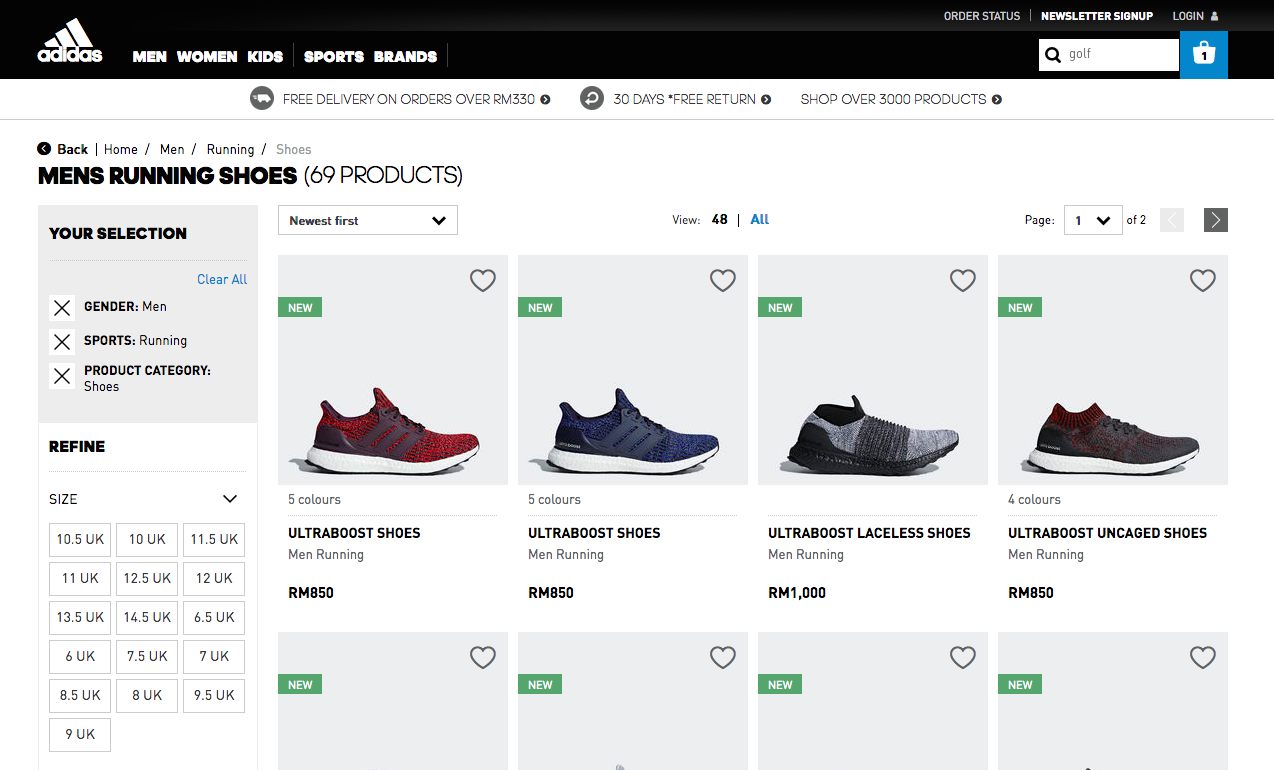Here is a cleaned-up and detailed caption for the described image:

---

Screenshot from the Adidas store website showcasing a variety of men's running shoes. At the top of the page is a black header featuring the Adidas logo and navigation tabs labeled "Men," "Women," "Kids," "Sports," and "Brands." On the right side of the header, there is a search bar alongside tabs for "Order Status," "Newsletter Sign-Up," and "Log In."

Below the header, a subheader announces, "Free delivery on orders over RM330," "30 days free return," and "Shop over 3,000 products." 

Further down, navigation breadcrumbs indicate the user is browsing: "Back > Home > Men > Running Shoes." A grey box on the left summarizes the current selection: "Gender: Men," "Sports: Running," and "Product Category: Shoes," along with size refinement options.

Displayed prominently are four products. The first is a red Ultraboost shoe with black trim, priced at RM850. Next is a blue Ultraboost shoe with darker blue trim, also priced at RM850. The third product is a gray Ultraboost Laceless shoe, appearing to be made from felt-like materials, priced at RM1000. The last product is a black Ultraboost Uncaged shoe, priced at RM850.